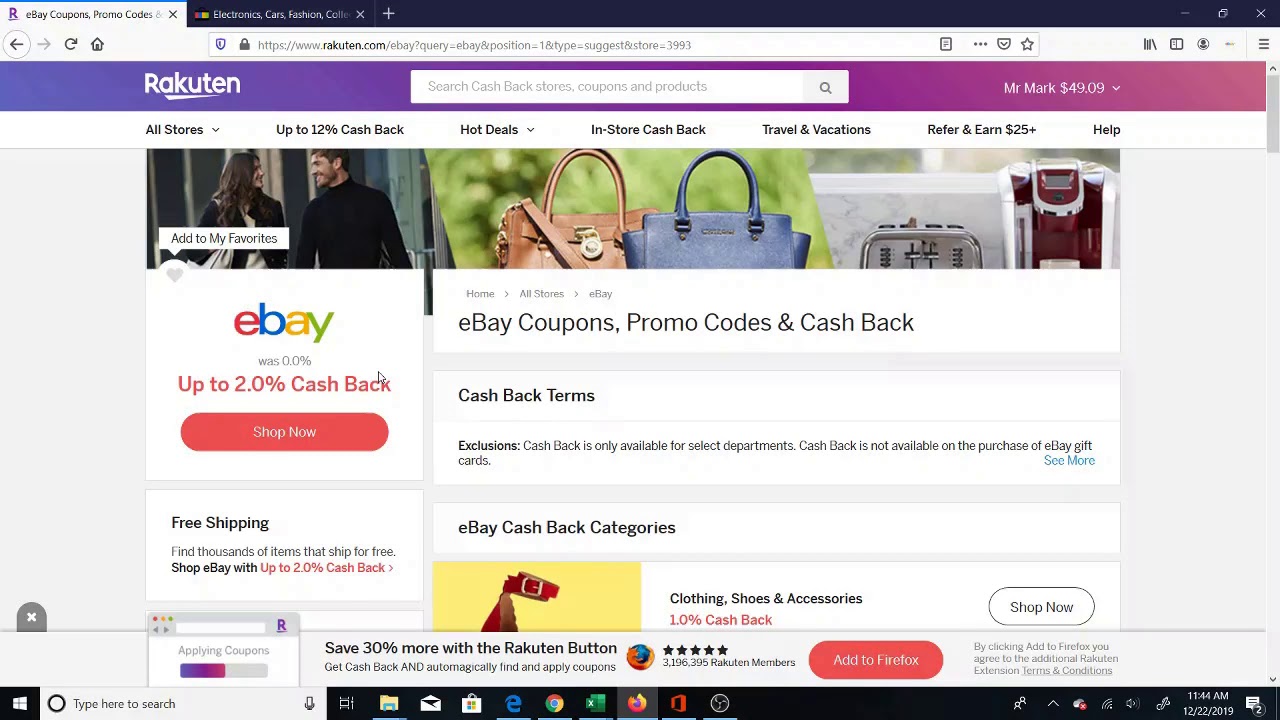This detailed descriptive caption describes an image that is a full-color screenshot of a computer's web browser and desktop environment. The screenshot was taken at 11:44 a.m. on December 22, 2019. The taskbar at the bottom of the screen reveals that the user has multiple applications open, including Microsoft Edge or Explorer, Google Chrome, Microsoft Excel, Mozilla Firefox, Adobe Acrobat (or what appears to be), and a Windows File Explorer folder. Additionally, the taskbar shows that the user has two unread emails. The browser captures the main page of the Rakuten website, www.rakuten.com, where the user is logged in as Mr. Mark, who has a current balance of $49.09 available for spending. The browser interface includes several navigation tabs, such as “All Stores,” “Up to 12% Cash Back,” “Hot Deals,” “In-Store Cash Back,” “Travel and Vacations,” “Refer and Earn $25,” and “Help.” Below these tabs, an eBay advertisement is displayed, offering up to 2.0% cash back with an option to "Shop Now." Additionally, a banner on the webpage features two models smiling at each other with handbags prominently displayed as part of the promotional content.